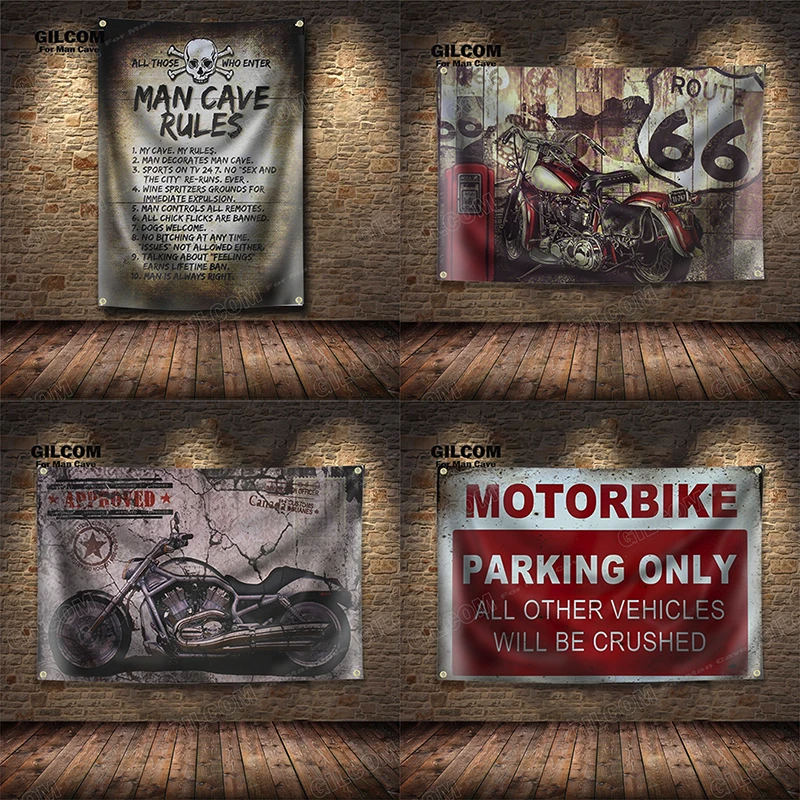In this image comprising four distinct sections, we observe the interior of a brick building featuring hardwood floors running vertically. Each section showcases a poster affixed to a wall composed of brown bricks. 

In the upper-left section, there's a poster with the headline "Gilcom for Man Cave," displaying the "Man Cave Rules." A skull and crossbones embellish the top, followed by various humorous rules such as "Man is always right" and "No chick flicks are banned." 

The upper-right segment includes a poster depicting a red motorcycle with a black seat under the title "Gilcom Route 66." 

In the bottom-left corner, another angle presents a black and silver motorcycle with an "Approved" label next to it. 

Finally, the bottom right features a red and white banner reading, "Motorbike Parking Only, All Other Vehicles Will Be Crushed."

This detailed image presents a coherent theme centered around a "Man Cave" adorned with motorcycle-related decor and humorous signage.